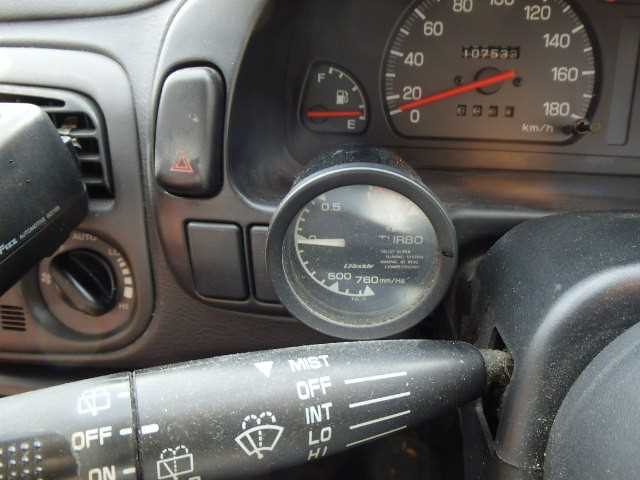The photograph showcases a detailed view of an automobile's dashboard and its instrument panel. The dashboard is predominantly dark gray, accented with clear white numbering and font. Centrally featured is the fuel gauge, distinguished by a white font and an image of a gas pump, along with a red needle indicator. Adjacent to it is the speedometer, similarly marked with white numbers and a red needle. A notable black circular object protrudes from the instrument panel, marked with various numbers and a white arrow.

Beneath this, the turn signal stalk is visible, along with settings for wiper speeds. The edge of the steering wheel is partially captured, noticeably dusty and covered in dirt and debris, indicating wear and age. This dashboard employs an analog display, not a digital one. Additionally, part of the vehicle's air vents are visible on the dashboard. The overall image quality is somewhat grainy, adding a textured, vintage feel to the photograph.